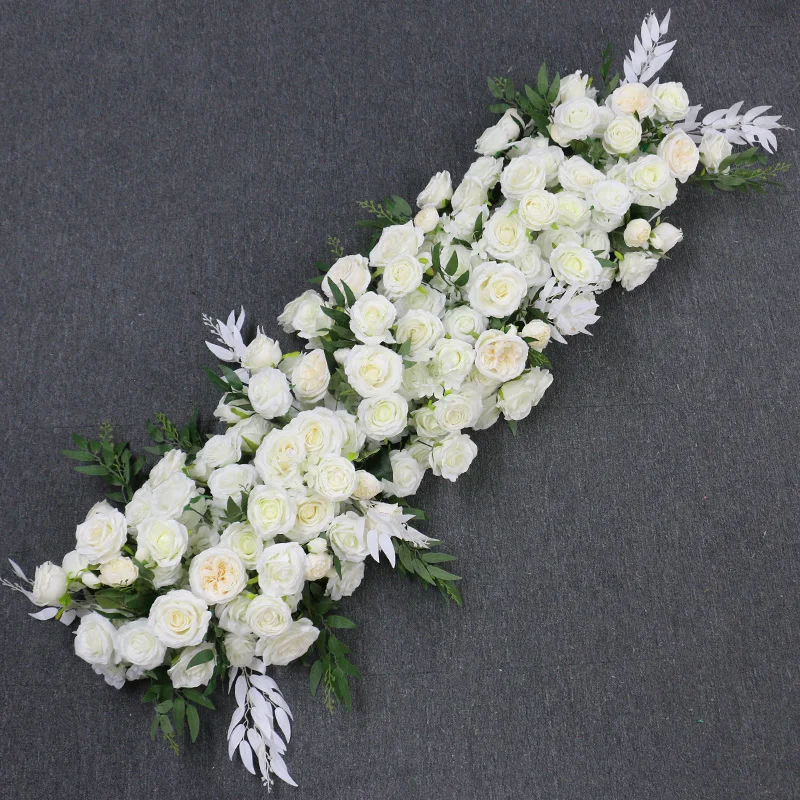The photograph showcases a long, narrow flower arrangement designed for a somber occasion, likely to be placed on a coffin. This elegant array features approximately three dozen pristine white roses, arranged in a diagonal line stretching from the bottom left to the top right corner of the image. Among the roses are slender green leaves, some of which have been artfully painted white, adding a unique texture and contrast to the composition. The background is a dark grey fabric, seemingly like a piece of cloth or even a t-shirt, providing a muted backdrop that enhances the arrangement's stark beauty. The overall effect is a sophisticated blend of natural and altered elements, creating a respectful and serene visual homage.